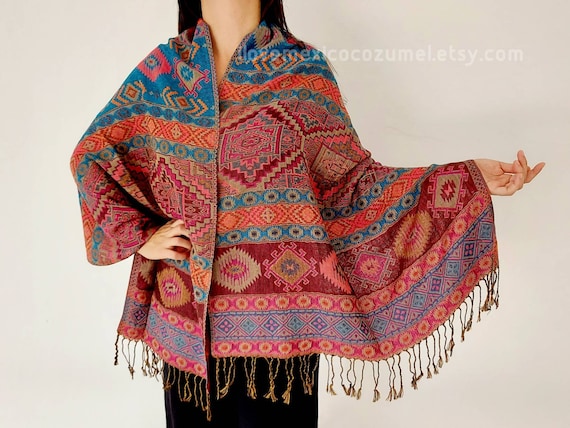This image features a model, with her head and face cropped out of the frame, standing against a white-gray background. The model, who has light-complected skin and dark brown hair, is dressed in black pants. Her left hand rests on her hip, while her right hand is extended outward. She is wearing a colorful poncho adorned with intricate geometric patterns. The poncho transitions from dark blue at the top into various designs featuring red, beige, and orange diamonds and rectangles, followed by a checkered pattern with red axes and diamonds interspersed with beige diamonds. Further down, the poncho exhibits a carpet-like design of interconnected red squares and diamonds, outlined in beige, and is finished with tan fringes at the bottom. In the top right corner of the image, there's a watermark that reads, "I love Mexico Cozumel," followed by the text, "lovemexicocozumel.etsy.com." This photograph appears to be an advertisement for the poncho, marketed on Etsy.